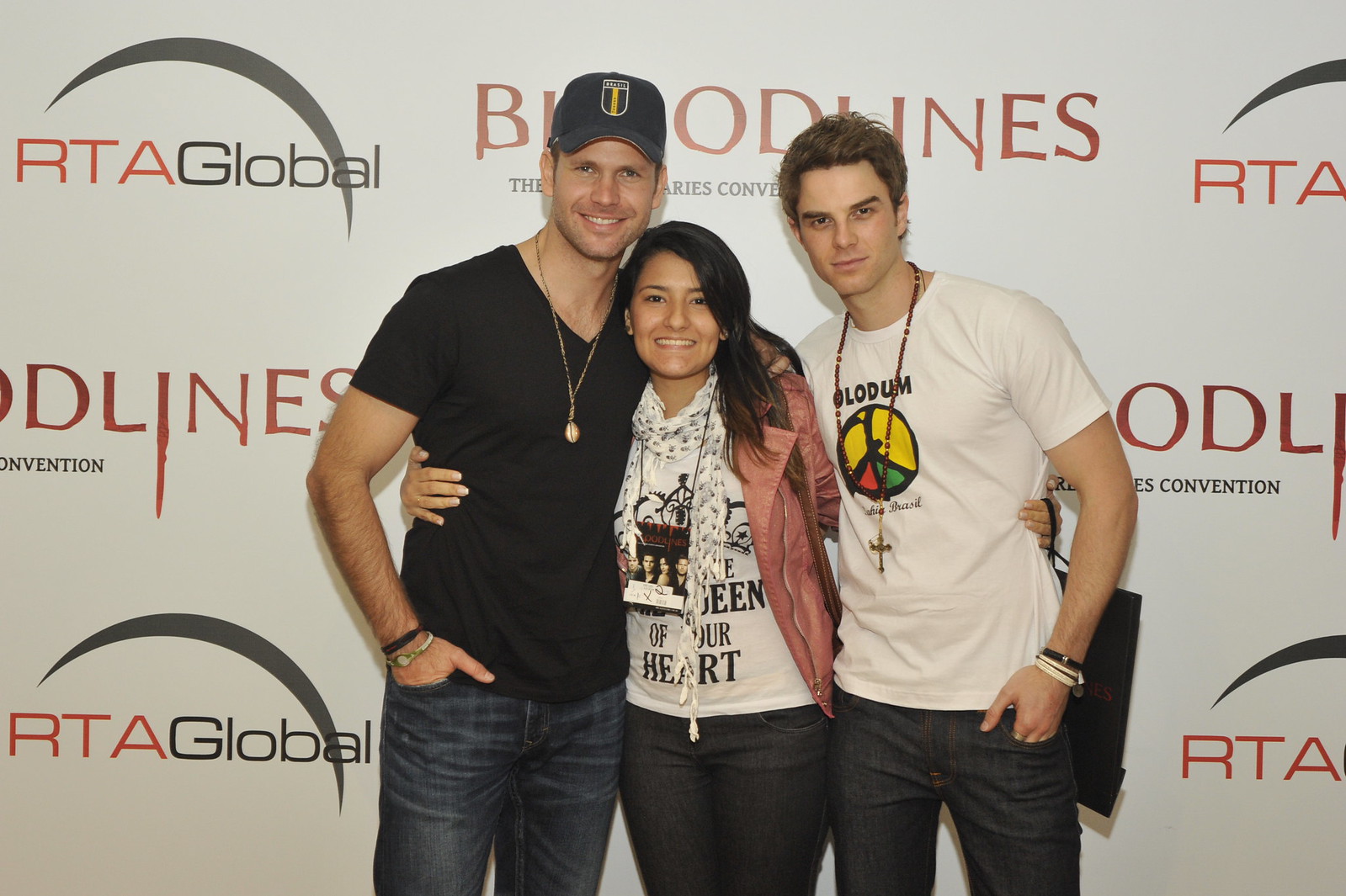The photograph features three individuals posing together in front of a branded backdrop at what appears to be a press event for the Bloodlines: The Vampire Diaries Convention, sponsored by RTA Global. The backdrop prominently displays the event's name and sponsor. From left to right, the group consists of a taller white man wearing a bluish baseball cap with a logo, a black v-neck short-sleeved t-shirt, and dark blue jeans. He has one hand tucked into his pocket and the other arm around his companions, smiling at the camera. In the center stands a woman with olive-toned skin, long brown hair, a white t-shirt with "Queen of Your Heart" printed on it, jeans, and a pink coat. She has a press badge hanging around her neck. To the right is another white man dressed in a white t-shirt, dark jeans, and a cross necklace. He presents a serious, smoldering look to the camera. Both the men flank the woman, collectively radiating a mix of casual style and confident poise against the backdrop highlighting the convention and its sponsors.